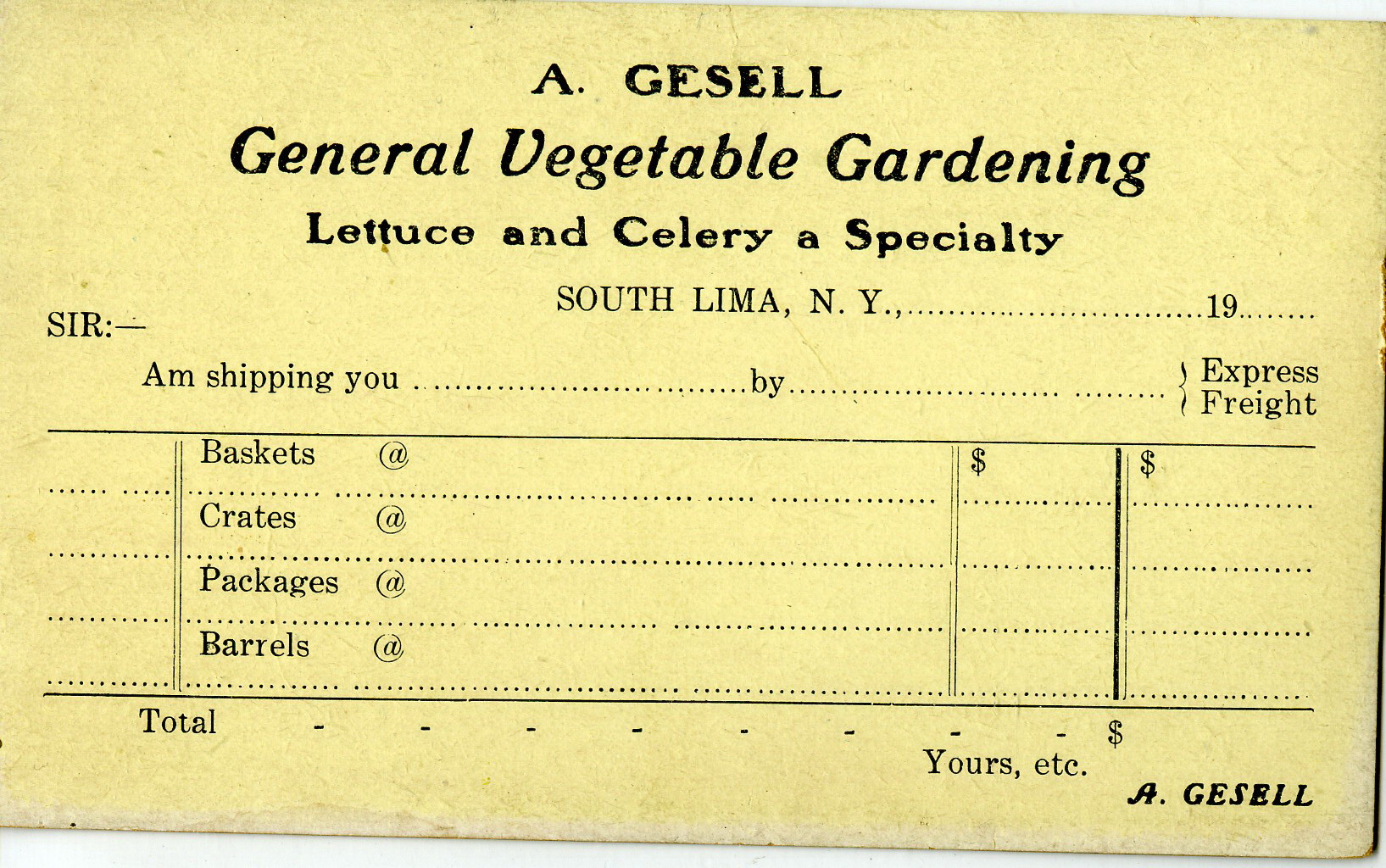This antique invoice from A. Gessell General Vegetable Gardening, specializing in lettuce and celery, is set on a horizontal, rectangular sheet of beige paper with black type lettering. Originating from South Lima, New York, the invoice prominently displays the company name and specialization at the top. Beneath that, it includes a line for filling in the year, starting with "19__". The form reads "Am Shipping You ___ by ___ Express Rate" and features a table for itemized entries, listing baskets, crates, packages, and barrels, sectioned off with vertical and horizontal lines for totals. The design suggests it was used for shipping vegetable orders with an area for monetary totals, presumably from around the early 20th century.